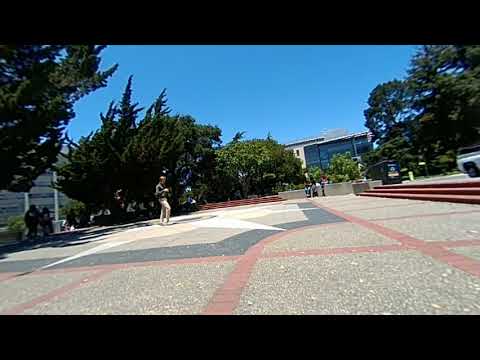This image captures a vibrant college campus scene centered around a wide, paved ground area featuring a white starburst design amidst aggregate concrete bordered by red brick tiles. The courtyard, set beneath a clear blue sky, leads to three brick steps that ascend to a higher level of flat ground. Flanking the walkway are lush green trees on both sides, providing shady spots where several individuals are seen standing and conversing, adding a sense of community to the setting. Ahead, a distinctive black building with reflective glass panels rises, suggesting a multi-story academic or administrative facility. A person dressed in tan pants, a green sweatshirt, and a backpack is walking across the starburst on the ground, adding a human element to the scene. In the distance, a white truck with construction racks and additional people underline the active and bustling atmosphere typical of a college campus.